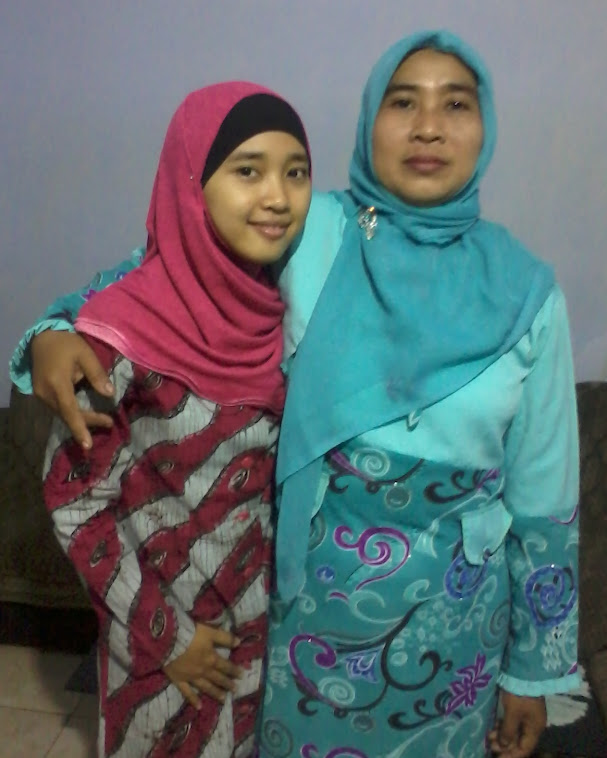In this indoor photograph, two women, likely of Middle Eastern or Islamic descent, are standing side by side, facing the camera and showcasing a close, affectionate bond. Each woman is adorned in traditional Islamic attire, with their heads covered by headscarves but their faces exposed. The younger woman on the left, who appears to be around 16 or 17 years old, wears a maroon headscarf layered over a black under scarf, a maroon-pink top scarf, and a horizontally striped long robe in maroon and white hues. She holds her right hand at her side, presenting a serene demeanor. The older woman on the right is dressed predominantly in green, with a blue headdress styled in a kerchief-like fashion, gracefully layered over a light blue-green top and a bottom that features flowing curves in purple, black, and blue. This woman has her right arm wrapped lovingly around the younger one’s shoulder while keeping her left arm down by her side. The backdrop is a simple gray wall, and the floor beneath them is tan, which emphasizes the vibrant colors of their clothing. One woman smiles more than the other, highlighting a slight difference in their expressions. Overall, the vivid, flowing colors paired with their tender pose create a warm, harmonious image of family or friendship.